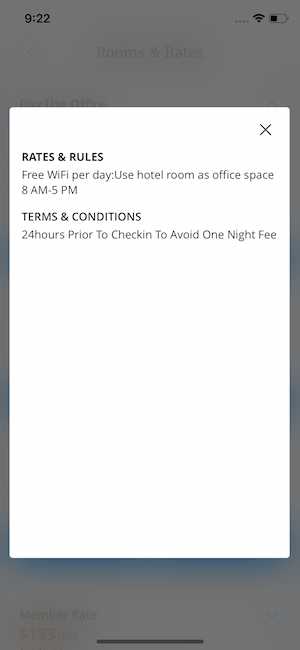The image features a screenshot from a smartphone display. In the foreground, there is a pop-up menu with a white background and black text, centered on the screen. The menu details various options, including "Rates and Rules," "Free Wi-Fi per Day," and "Use Hotel Room as Office Space, 8 a.m. to 5 p.m." Below these options, it mentions the "Terms and Conditions," specifically stating that cancellations must be made "24 hours prior to check-in to avoid a one-night fee."

The main app page is visible in the background, with a slightly transparent overlay. This background features a dark color scheme. At the top of this main page, the text "Rooms and Rate" is written in black. There is a blue back button located on the top left corner of the screen. Below this, black text reads "Day Use Office."

At the bottom of the image, there is additional text in black, stating "Member Rate, Madison Territory," followed by an orange-colored price, "Madison Territory U.S. Dollars," with "USD" written in black.